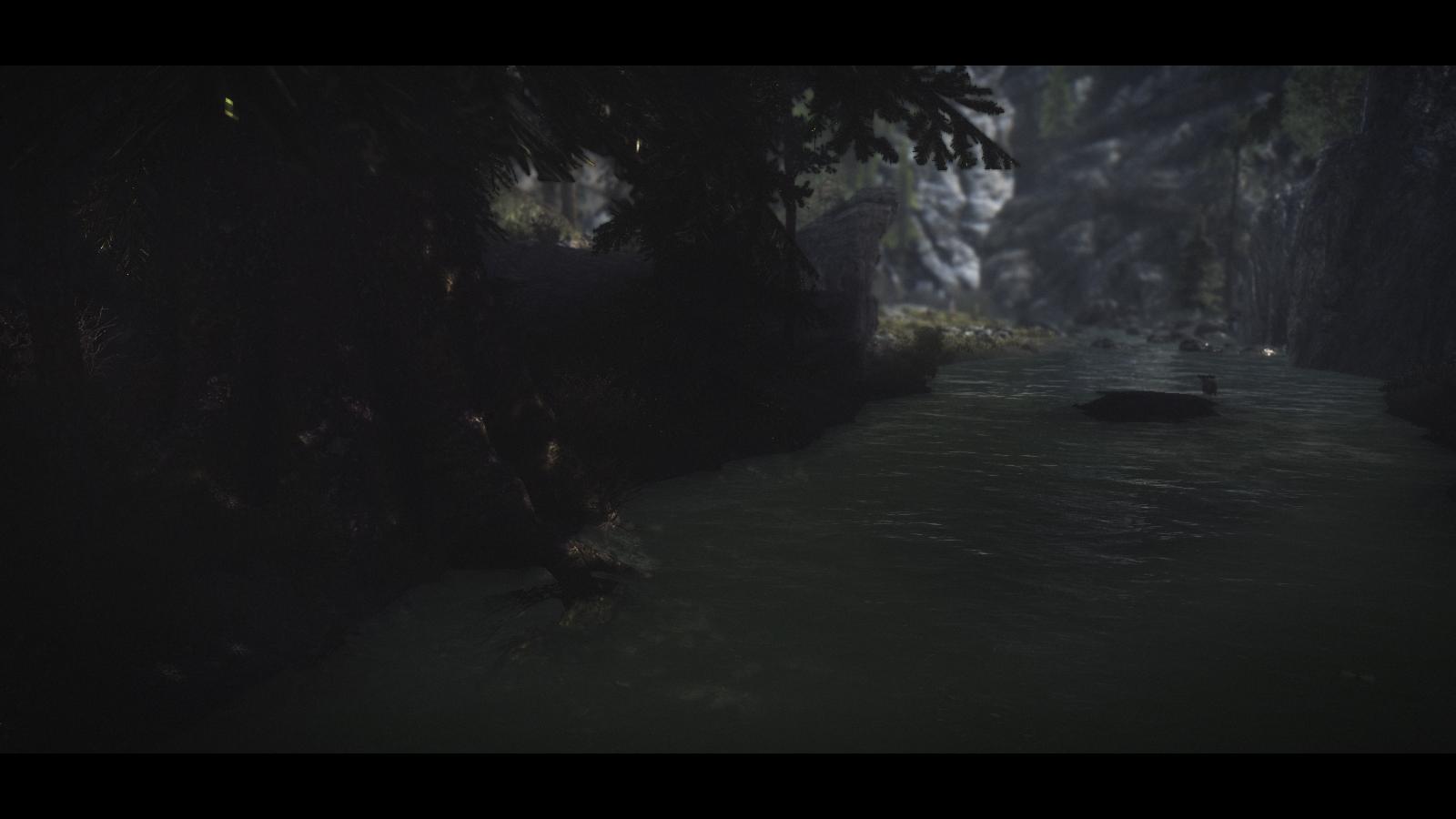This rectangular image is of low quality, characterized by its dark and blurry nature. At the top and bottom, there are black bars extending horizontally across the entire width of the photo. Despite the lack of clarity, a body of water is discernible on the right side, displaying faint lines that suggest the presence of waves, with the water appearing gray. An indistinct object or structure is seen on the water's surface, though it is too blurred to identify clearly. In the upper left corner, the silhouette of trees and leaves is visible, accompanied by an assortment of green plants in the background. The overall scene exudes a murky, obscure ambiance.